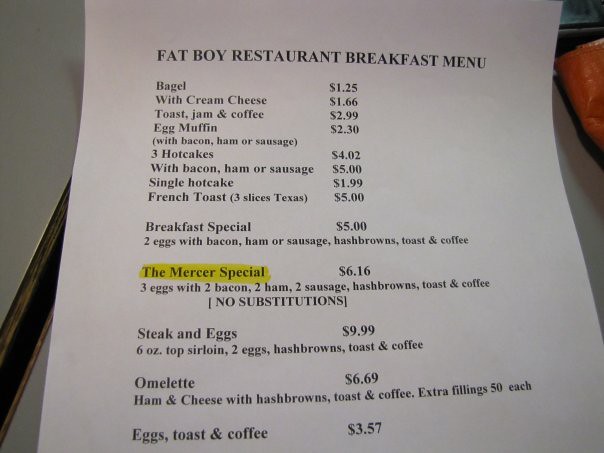This photograph captures a printed breakfast menu from the Fat Boy Restaurant, presented on a simple white piece of copy paper. At the top, the menu title "Fat Boy Restaurant Breakfast Menu" is displayed in bold, black font in a single line. 

The menu is divided into a la carte items and specials:

**A la carte items:**
- Bagel: $1.25
- Bagel with Cream Cheese: $1.66
- Toast, Jam, and Coffee: $2.99
- Egg Muffin with Bacon, Ham, or Sausage: $2.30
- Three Hot Cakes: $4.02
- Three Hot Cakes with Bacon, Ham, or Sausage: $5.00
- Single Hot Cake: $1.99
- French Toast (Three slices of Texas Toast): $5.00

**Specials:**
- Breakfast Special: $5.00
  - Includes two eggs with bacon, ham, or sausage, hash browns, toast, and coffee
- Mercer Special: $6.16
  - Features three eggs with two bacon, two ham, two sausages, hash browns, toast, and coffee (no substitutions)

Additional items listed but not detailed with prices include:
- Steak and Eggs
- Omelette and Eggs
- Toast and Coffee

Each item is meticulously detailed, providing customers with a clear choice of breakfast options offered at this classic diner.